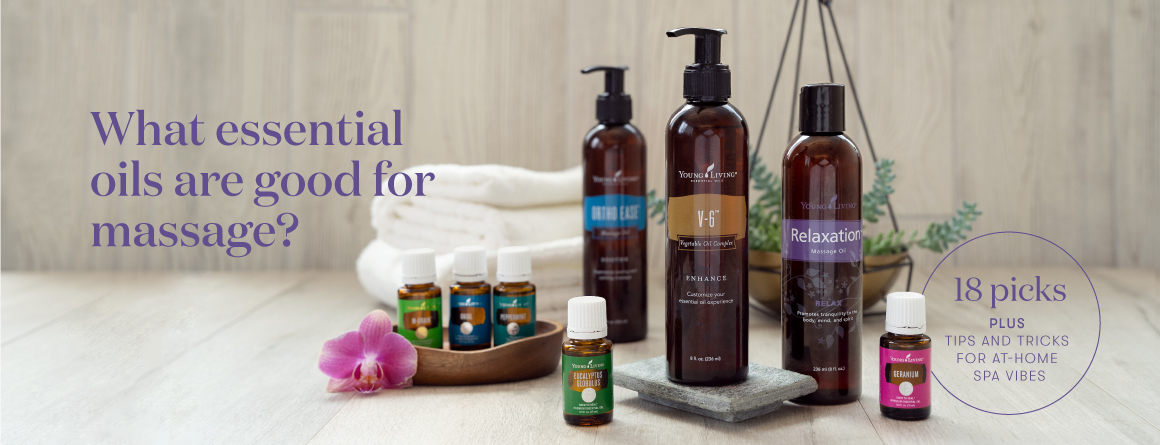This color photograph exudes a spa-like ambiance, showcasing a selection of essential oils perfect for massage. The backdrop features a whitewashed wooden surface with stacks of plush, white towels and a hanging plant pot brimming with succulents, adding a touch of greenery and tranquility to the scene. 

In the foreground are three large, dark brown bottles with black caps, arranged from left to right. The leftmost bottle and the central bottle are equipped with pump dispensers, donned with blue and orange labels respectively, with the central bottle labelled "V-6." The rightmost bottle features a purple label inscribed with "Relaxation," and has a standard black cap without a pump. The central bottle is also placed on a small gray stone pedestal, seemingly a soap dish.

Flanking the larger bottles are five smaller, similarily hued vials with white caps. Two of these smaller bottles are positioned at the front—one with a green label and the other with a pink label. The remaining three small bottles rest in a wooden basket to the left of the blue-labeled tall bottle, bearing green, blue, and aqua labels.

Adding to the relaxing visual, a delicate pink orchid blossom lies in front of the wooden basket. Supplementary text in purple script enhances the spa theme: "What essential oils are good for massage?" on the left side, and "18 picks plus tips and tricks for at-home spa vibes" inside a circular outline on the right. The meticulous arrangement of elements in this image underscores the inviting and serene atmosphere of a perfect at-home spa setup.